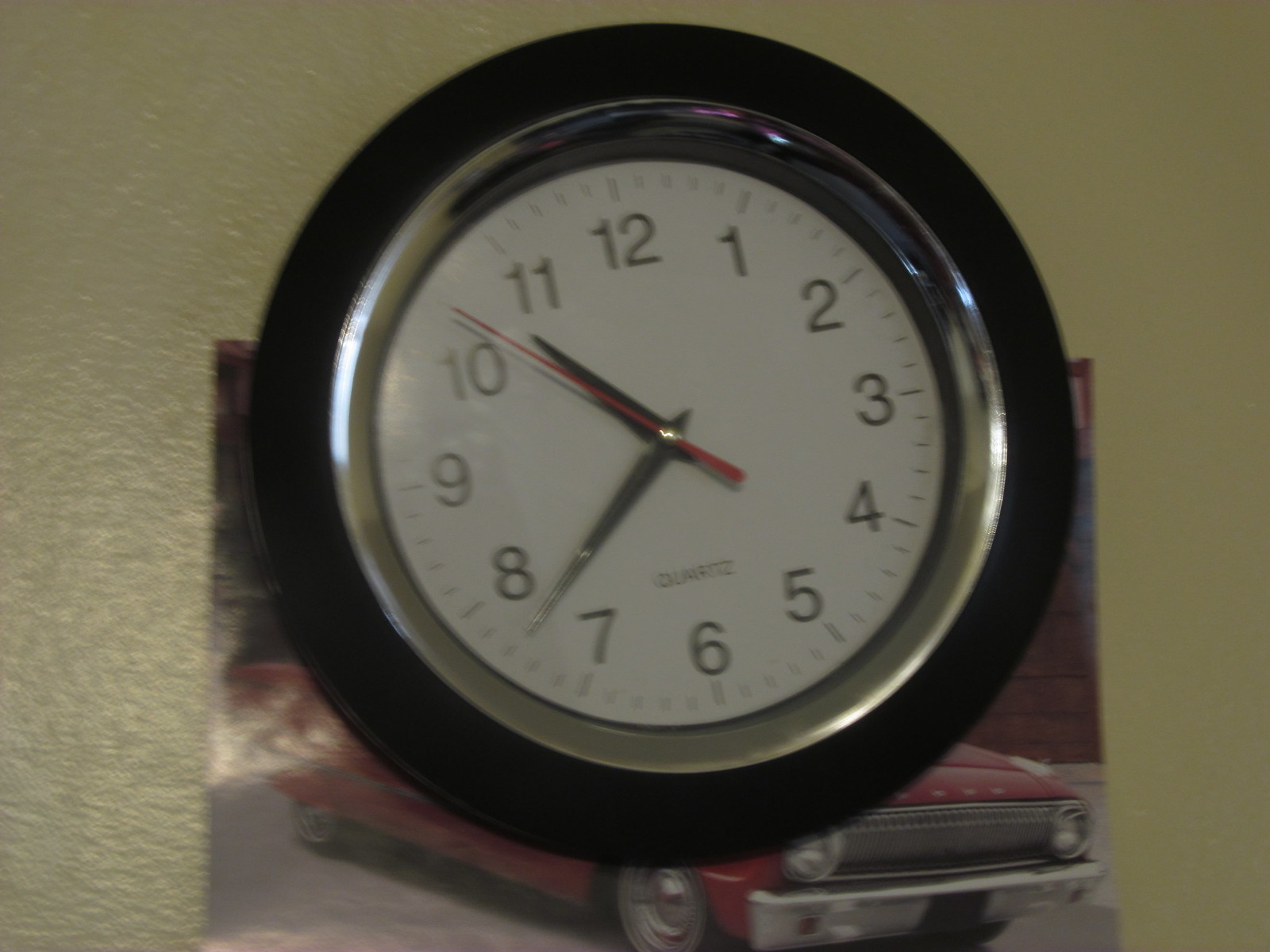This photograph captures an analog clock hanging on a textured, dimpled yellowish-brown wall. The clock is slightly tilted, about 10 degrees counterclockwise. It features a reflective grayish metal rim encircling a white dial with black numbers and a red second hand, alongside black hour and minute hands. The clock's time is precisely 10:38 and 52 seconds. Behind the clock, there's an image of a classic red American car, possibly a Ford or another 50s-60s model coupe. This image might be part of a calendar, although it's partially obscured by the clock, making the exact nature of the image speculative. The wall and the overlapping elements combine to create a vintage aesthetic, enhanced by the slight blur of the photograph.